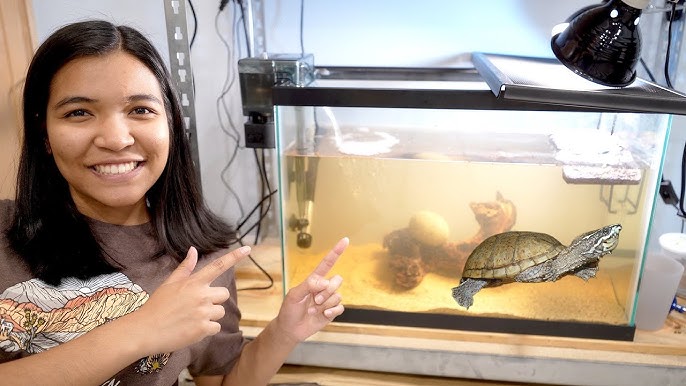This is a digitally altered photograph of a smiling young girl with fairly dark skin and long dark hair that falls past her shoulders. She is wearing a brown or grayish t-shirt featuring a mountain graphic illustration, and she is enthusiastically pointing with both hands towards an aquarium. The aquarium, which is set on a wooden shelf with metal supports, has a black base and top, and contains murky, yellowish water. A bright lamp mounted on the top right through a black rectangular screen shines down into the tank. At the top left, a transparent plastic box with cables is visible, running up along the wall. Inside the tank, there is sand at the bottom, and a piece of wood or rock sits at the center. Notably, an image of a small to medium-sized aquatic turtle with webbed feet has been superimposed in the bottom right area of the aquarium, giving it the appearance of swimming in the tank. The girl, who appears to be of Latina descent, is looking directly at the camera, exuding happiness and pride in the tank.